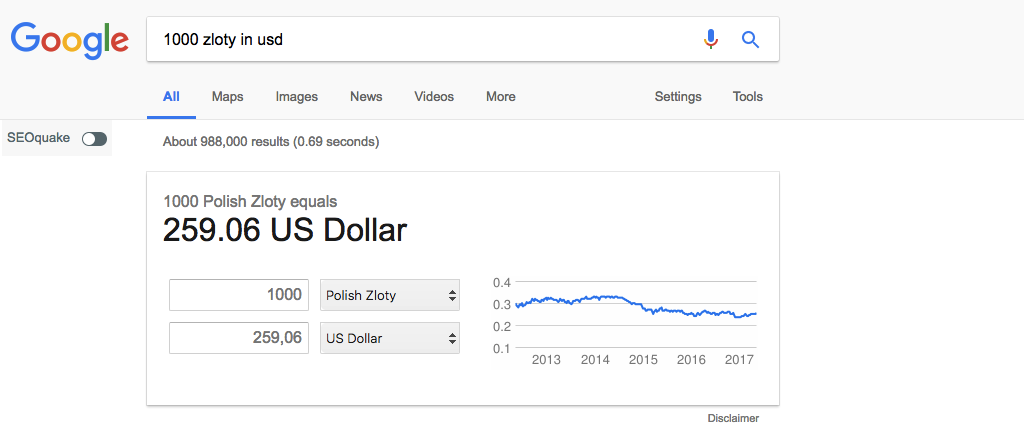The screenshot captures a Google search page. In the top left corner, the Google logo is displayed in its distinctive alternating colors: blue, red, yellow, blue, green, red. Centered below the logo is a search bar querying "1000 Zloty in USD," with a microphone icon and a magnifying glass search icon situated at the right end of the bar.

Immediately beneath the search bar, the selected "All" tab is highlighted among other search categories: Maps, Images, News, Videos, More, Settings, and Tools. To the left side, there is a slider button for SEO Quake, currently in the off position. Below these options, a brief search result summary indicates approximately 988,000 results in 0.69 seconds.

The main search result prominently displays the conversion rate: "1000 Polish Zloty equals 259.06 USD" and "1000 Polish Zloty to USD 259.06." Adjacent to this, on the right, is a graph illustrating the progression of this exchange rate from 2013 to 2017. At the bottom right of the screen, the word "disclaimer" is visible. This Google screenshot contains no images or photographic elements, and no people are present.